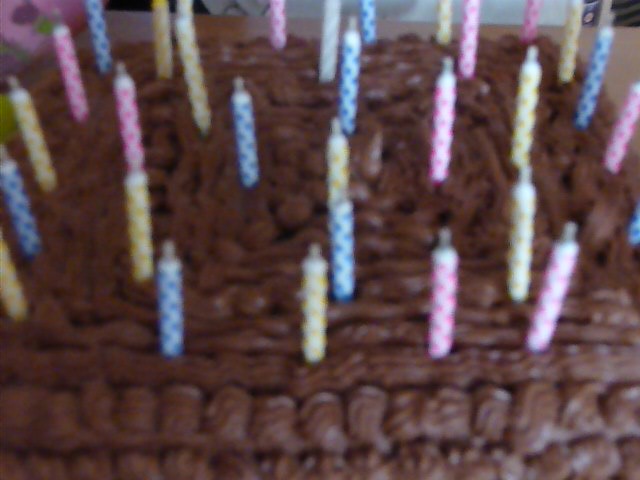This is a very blurry, grainy image of a large, homemade chocolate birthday cake. The cake, square in shape, is heavily frosted with thick, intricately piped chocolate icing featuring various swirling and geometric patterns, although the piping appears somewhat clumsy and uneven. Despite the photo's poor quality, it's clear that the cake is adorned with many multi-colored birthday candles that haven't yet been lit. These candles are predominantly white with vibrant polka dots and diamond patterns in blue, yellow, red, and pink, randomly distributed across the top of the cake. The cake itself dominates the frame and sits on what looks like a smooth, brown wooden table.